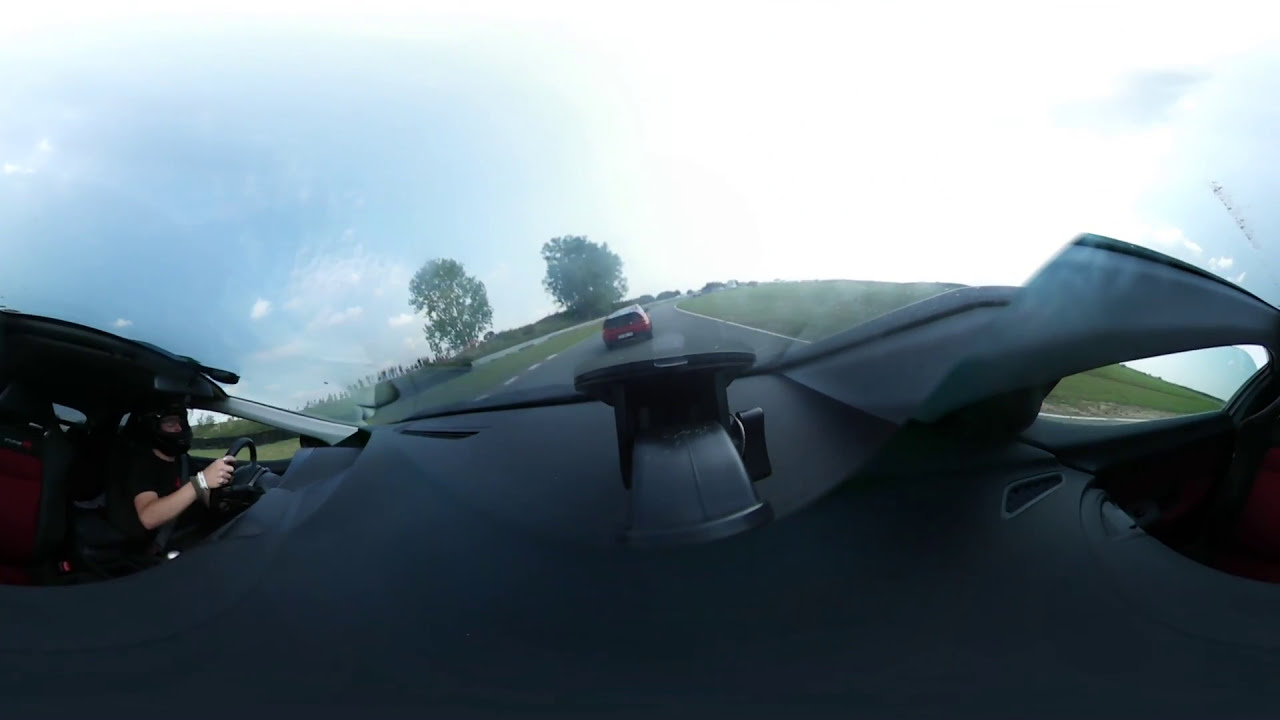The image captures the view from inside a car, looking through the front windshield on a sunny day with a partly cloudy blue sky. The focus is on the scene ahead, where a red car is driving in front on a black-paved road that appears to be an on-ramp. The road features a white stripe and is flanked by long grassy hills and a few trees, particularly noticeable on the left side.

Inside the car, the dashboard, which is black, is fully visible and has a piece of paper on it, the contents of which are unclear. To the left, there is another car seemingly attached, with a visible driver who appears to be a race car driver. This driver is wearing a helmet and a wristband, adding a unique element to the scene. Together, these details provide a comprehensive and intriguing snapshot of the moment.